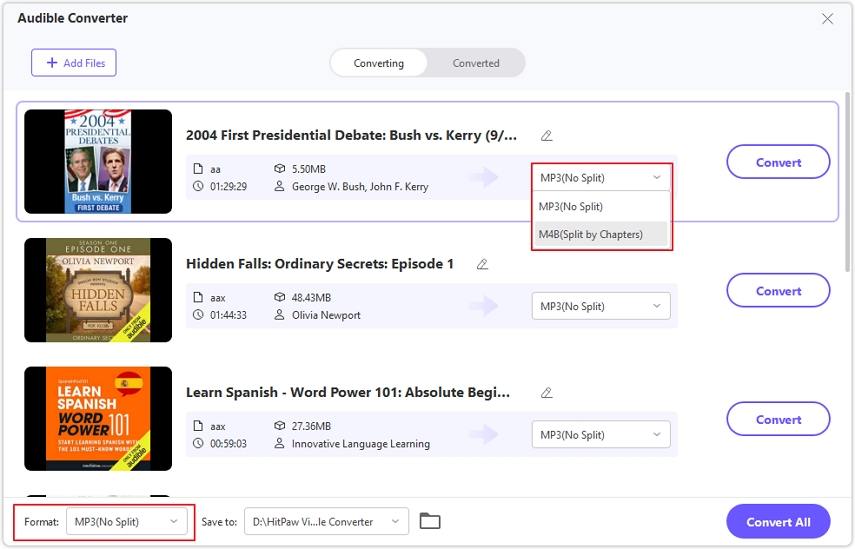The website features the title "Audible Converter" prominently in dark black text located in the upper left-hand corner. Below the title is an "Add File" section for users to upload files. The central part of the webpage, highlighted in light gray, has tabs labeled "Converting" and "Converted," with "Converting" currently highlighted.

The body of the webpage features a white background displaying several items listed for conversion, each with an accompanying image and descriptive text. The first item is labeled "2004 Presidential Debates: Bush vs. Kerry," featuring a black background with text indicating it pertains to the first presidential debate in 2004 between George Bush and John Kerry. There is a red box within this section that provides various conversion options, including MP3, MP3 split, and more. Each option is presented with its own white and purple-outlined button on the right side.

The second item listed is titled "Hidden Falls: Ordinary Secrets Episode One," with a cover image reflecting its theme. The third item, with an orange cover and titled "Learn Spanish," contains the text "World Power" underneath.

For users wishing to convert all displayed files simultaneously, there is a prominent solid purple "Convert" button located to the right. Additionally, a red box at the bottom indicates the selected format as MP3 with no split option.